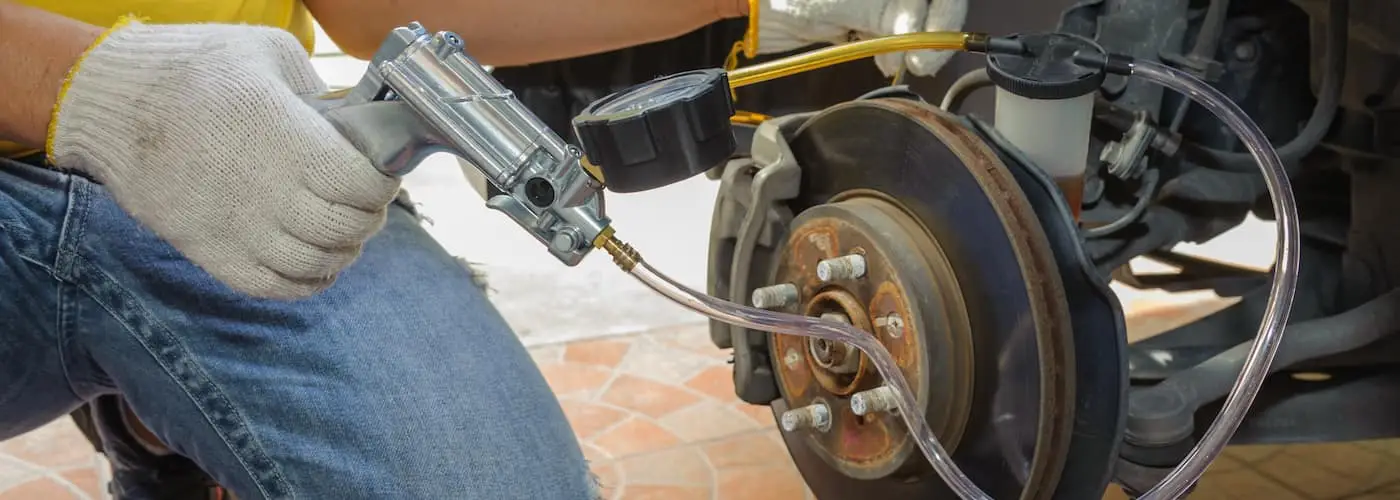The image captures a close-up scene of a mechanic, wearing jeans and white gloves with yellow rims, intently working on a vehicle's brake system. The mechanic is kneeling on terracotta-tiled ground, focusing on the brake pads with the tire removed, revealing the intricate mechanics beneath. He is holding a silver-colored tool connected to a hose, which routes fluid—likely brake fluid—into the brake assembly. This hose extends through a plastic container, leading to a yellow hose attached to a meter for monitoring or measurement purposes. The brake components show signs of wear with visible rust, particularly around the dark-colored, gear-like elements secured by bolts. The entire wheel is disassembled, highlighting the detailed maintenance process being conducted.